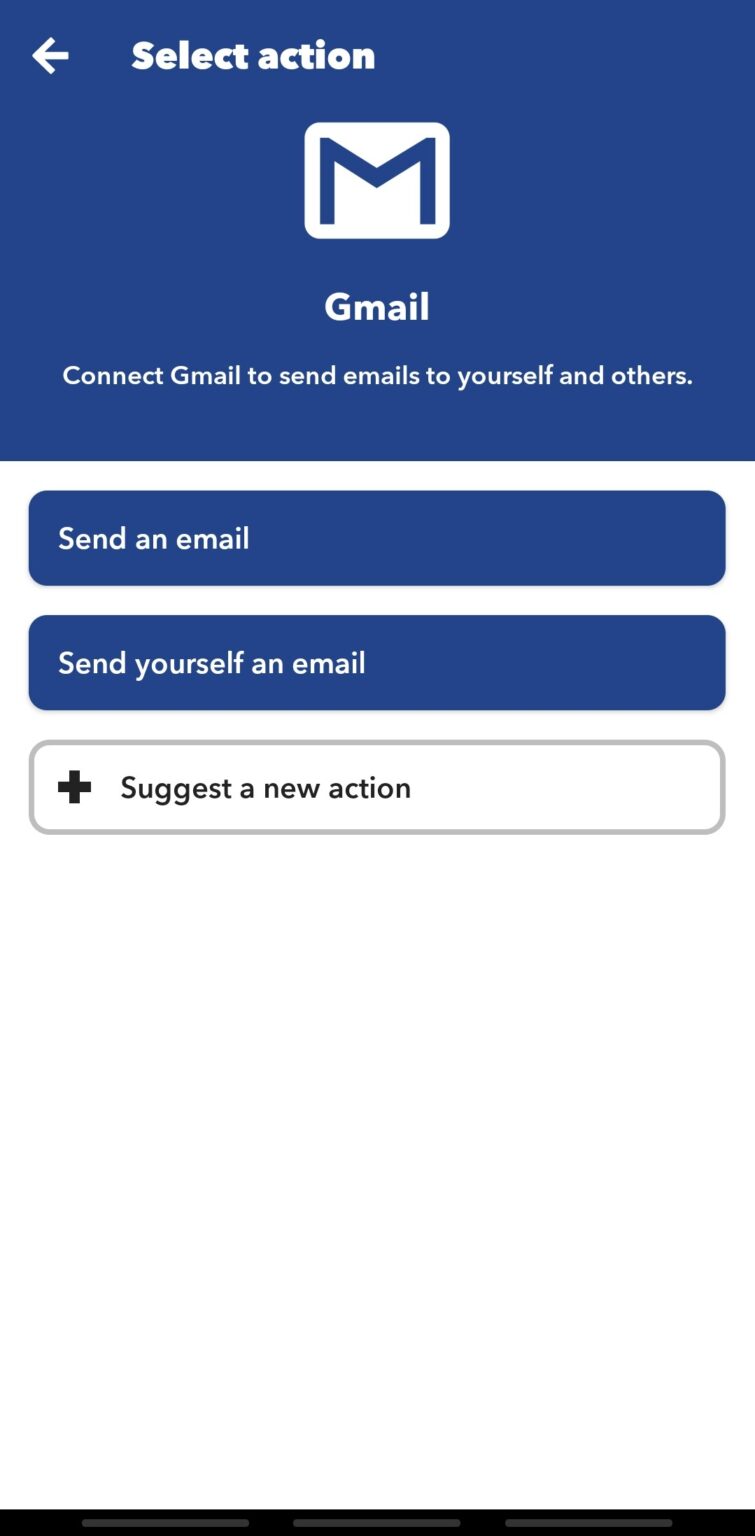The image features a predominantly dark blue interface section at the top. On the top-left corner, there is a white arrow pointing to the left. Immediately to the right of the arrow, the text "Select Action" is displayed. Below this header, there is a white rectangle with a large blue "M" in the center, representing Gmail. Underneath the "M," the text reads "Gmail." Following this, there's a descriptive line stating, "Connect Gmail to send email to yourself and others."

Further down, there is a blank area followed by a smaller blue rectangle, which says "Send an email." Below this, another similarly sized blue rectangle is labeled "Send yourself an email." The final selectable option is a white rectangle outlined in blue, which features a plus sign on the left and the text "Suggest a new action."

Towards the bottom of the image, there is a substantial amount of empty space. At the very bottom, a black horizontal line extends across the entire width of the interface, from left to right.